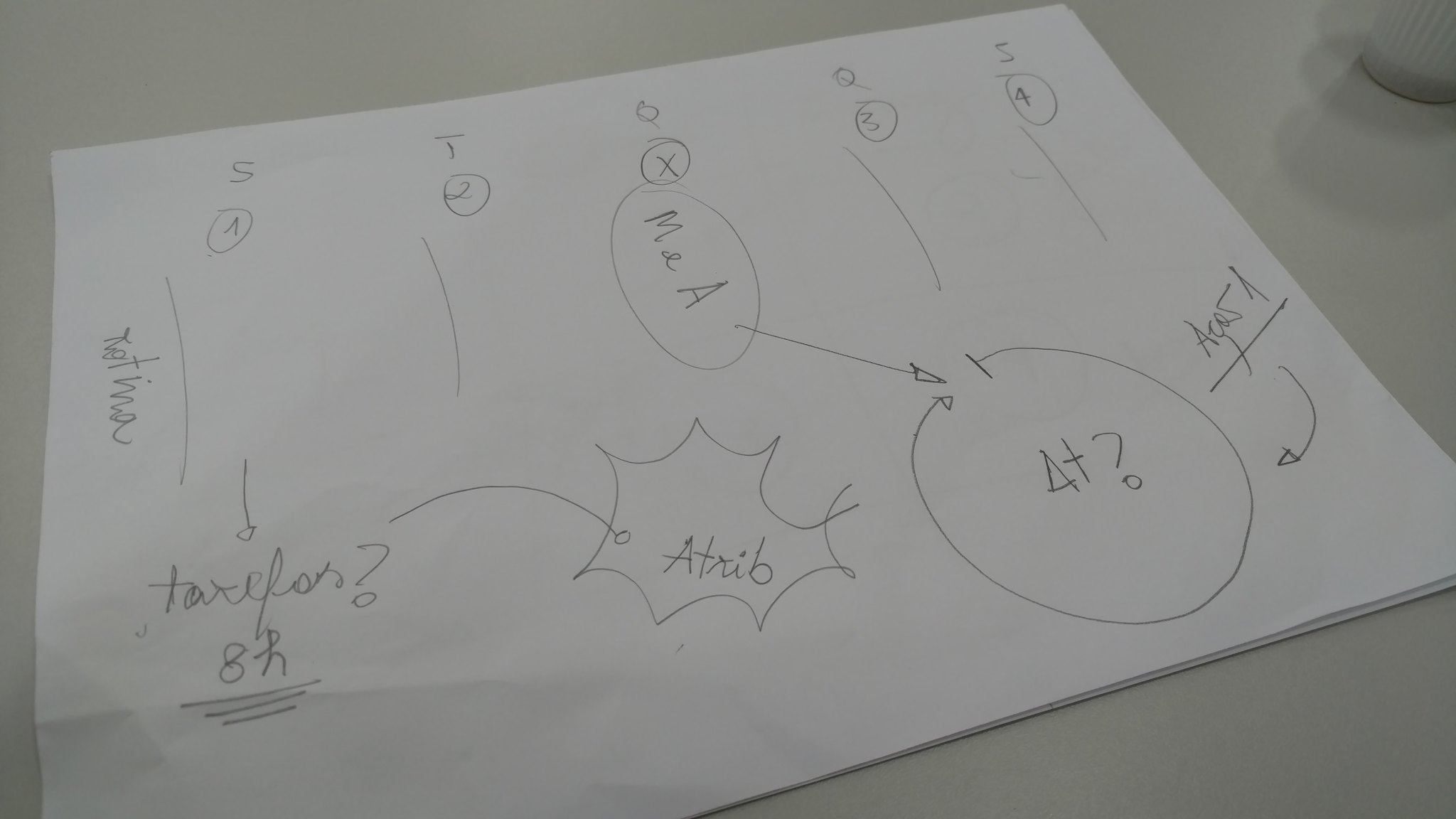The image features a sheet of paper resting on a white tabletop. The paper contains a hand-drawn diagram with various annotations, including words, letters, and numbers. Among the notations are phrases such as "me and A," "delta T?" and "Taylor's 8 hours," followed by "trib." Mathematical expressions like "A cosine A" are also present, suggesting the content is related to STEM subjects, possibly mathematics or science. The text and drawings appear to be penciled in.

In the background, a white object, which could be either a cup or a salt shaker, is slightly visible. The poor indoor lighting casts shadows of both the cup and the paper on the table. No additional objects or details are present in the image besides the paper and the background item.